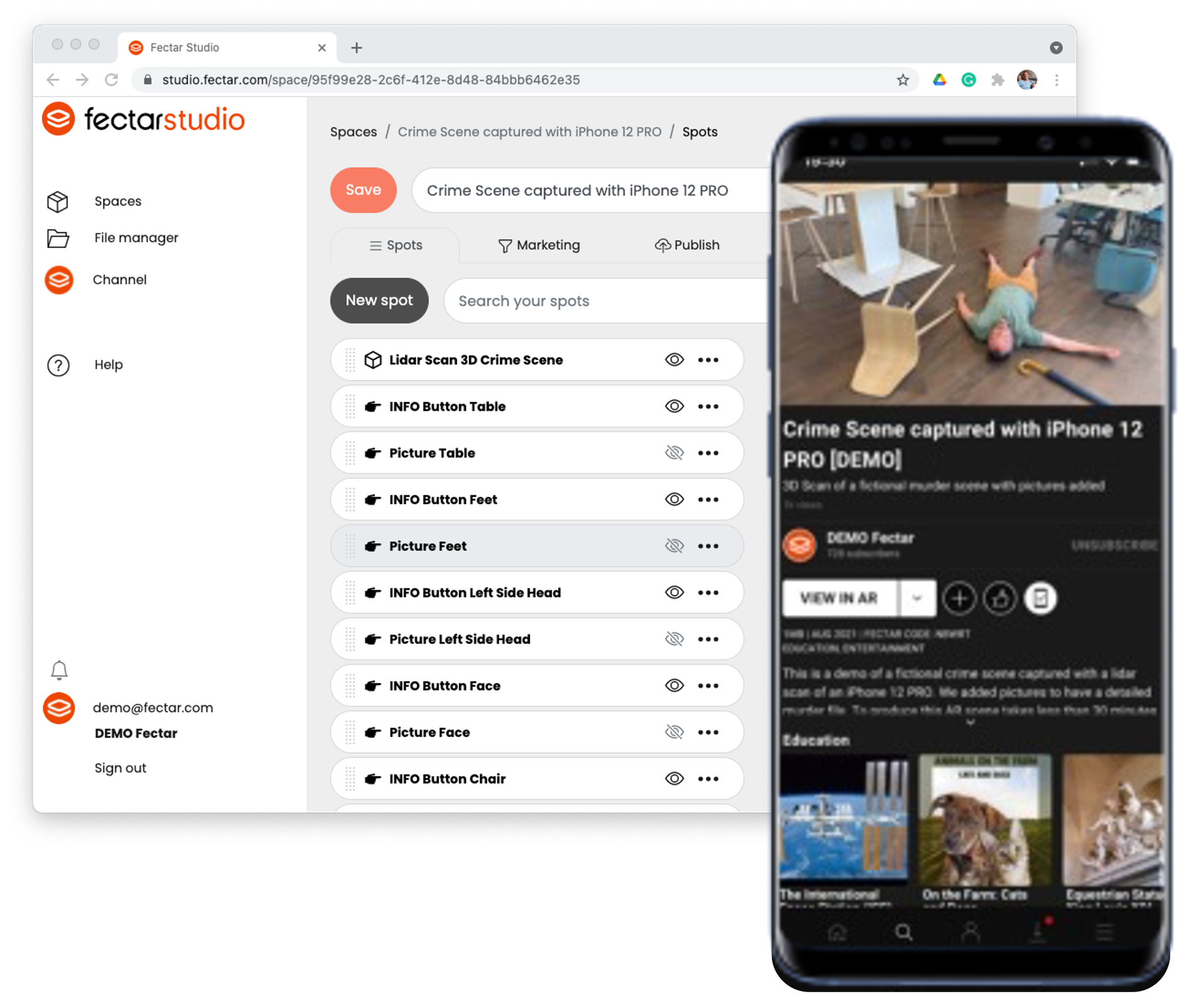This screenshot showcases a web page designed by Vector Studios. At the top of the page, there is a web bar, beneath which is a left-hand side white navigation panel listing several options including 'Spaces,' 'File Manager,' 'Help,' and a 'Demo' option at the bottom.

The main portion of the screen, occupying the right two-thirds, displays an image of a cell phone capturing what appears to be a crime scene. A label beneath the image reads "Crime Scene Captured with iPhone 12 Pro Demo." Several interactive options accompany this image, allowing users to explore various aspects of the crime scene.

Behind the central image, there is a gray box with several selectable options including "Spaces / Crime Scene Captured with iPhone 12 Pro," and sub-options such as "Save the Crime Scene Captured with iPhone 12," "Search Your Spots," "New Spots," and "LIDAR." Underneath these, more detailed interactive choices are listed such as "LIDAR Screen," "LIDAR Scan," "3D Crime Scene," "Info Button," "Table," "Picture Table," "Info Button," "Feet," "Picture Feet," "Info Button," "Left Side Head," "Left Side Picture," "Left Side Head Button Info," "Face," "Picture Face," and "Info Button." These appear to provide specific views and data points related to the crime scene imagery, potentially offering a variety of perspectives and in-depth details for analysis.